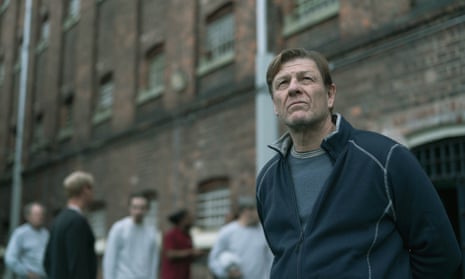The photograph depicts an older Caucasian man, possibly in his late fifties, standing prominently in the right quadrant of the image. He has light brown hair, a slightly wrinkled face, and fair skin. His expression is neutral, with squinted eyes and a slight frown, as he looks upward. He is dressed in a navy blue jacket with green piping over a light blue shirt. Behind him stands a brick building composed of red and grayish bricks, accentuated by green highlights around the windows and doors. This building, which may be an apartment complex, features metallic-looking steel pillars and gated or fenced-in windows. Five additional, blurry figures can be seen in the background, positioned over the man's right shoulder to the left of the photo. Among these figures, two are wearing long-sleeved white shirts, one is dressed in red, another in black, and the fifth one is in a gray long-sleeved shirt. The setting appears orderly, with clear lighting, but the exact expressions and details of the background figures remain indistinct.